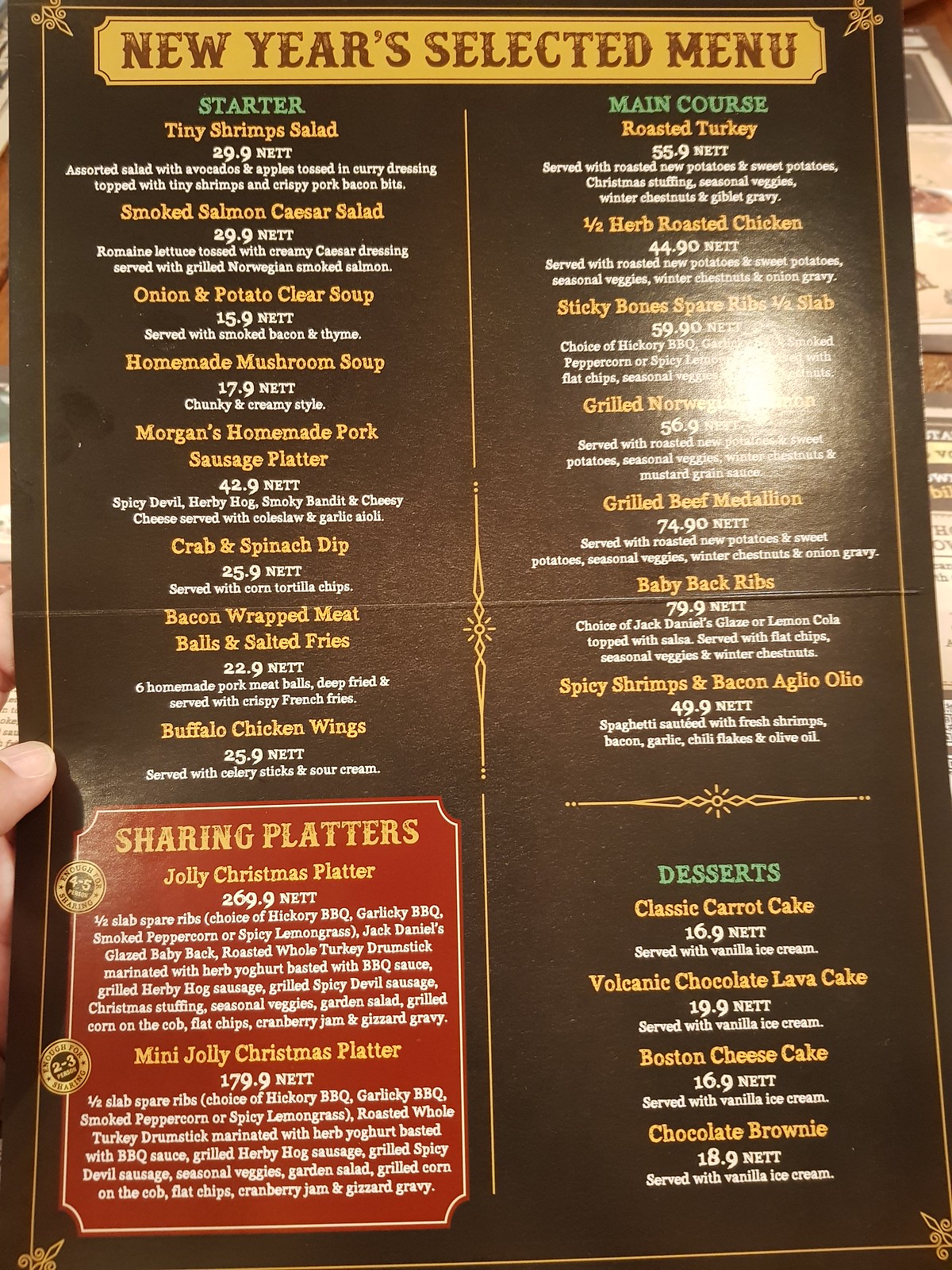**New Year's Selected Menu**

**Starters and Appetizers:**
- Tiny Shrimp Salad: 29.9 net
- Smoked Salmon Caesar Salad: 29.9 net
- Onion and Potato Clear Soup: 15.9 net
- Homemade Mushroom Soup: 17.9 net
- Morgan's Homemade Pork Sausage Platter: 42.9 net
- *Morgan's Homemade Pork Sausage Platter* (duplicate entry, same price)
- Crab and Spinach Dip: 25.9 net
- Bacon-Wrapped Meatballs with Salted Fries: 22.9 net
- Buffalo Chicken Wings: 25.9 net

**Sharing Platters (in a red bubble):**
- Jolly Christmas Platter: 269.9 net
- Mini Jolly Christmas Platter: 179.9 net

**Main Courses:**
- Roasted Turkey: [Price not provided]
- Half Herb-Roasted Chicken: [Price not provided]
- Sticky Bones Spare Ribs (Half Slab): [Price not provided]
- Grilled Norwegian Something: [Price not provided]
- Grilled Beef Medallion: [Price not provided]
- Baby Back Ribs: [Price not provided]
- Spicy Shrimps and Bacon Agiolo: [Price not provided]

**Desserts:**
- Classic Carrot Cake
- Volcanic Chocolate Lava Cake
- Boston Cheesecake
- Chocolate Brownie

Enjoy a delightful selection of our mouth-watering starters, main courses, and desserts to celebrate this New Year's occasion.